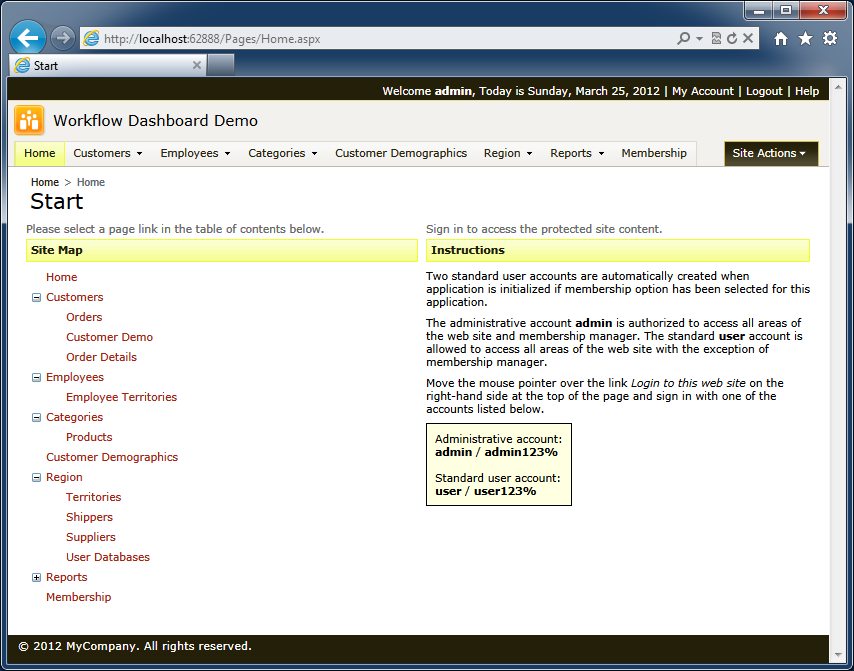The image, a screenshot of a dashboard interface, is displayed within a Microsoft Windows window. At the top, a URL containing "localhost" is visible, indicating a locally hosted web application accessed via Internet Explorer. The browser tab is open to a website that features a prominent black bar across the top of the window. 

Toward the middle-right of this black bar, the text reads "Welcome Admin. Today is Sunday, March 25, 2012," followed by "My Account," "Logout," and "Help" buttons aligned to the right. Below the black bar, there is a gray navigation bar that spans the width of the page. On the far left, it reads "Workflow Dashboard Demo."

This gray bar includes various navigation buttons arranged horizontally: Home, Customers, Employees, Categories, Customer Demographics, Region, Reports, and Membership. Notably, the Customers, Employees, Categories, Region, and Reports buttons feature drop-down menus for additional options.

Below this navigation bar, the layout transitions into a two-column structure. The left sidebar contains navigational elements or options, while the right side displays a text passage, likely providing detailed content or instructions related to the workflow dashboard.